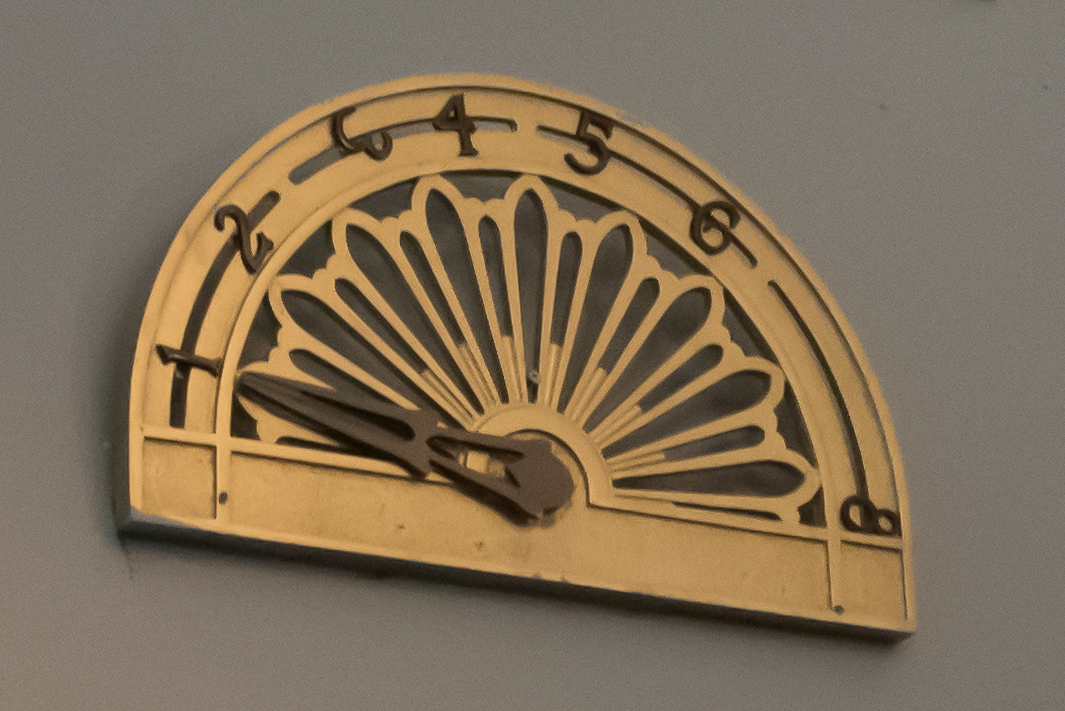A vintage pre-digital elevator indicator is showcased in this image. This classic timepiece-style design features a brass, segment-shaped dial reminiscent of an orange wedge, with a large clock hand-like brass pointer. The metal numbers encircle the dial, ascending from 1 to 8, although the number 7 is conspicuously absent. Notably, the number 3 is slightly skewed, leaning almost upside down but not quite. The darker, somewhat tarnished brass pointer currently indicates floor 1. The entire assembly, including the similarly colored numbers, is mounted against a pristine white wall, highlighting the antique aesthetic of the elevator indicator.